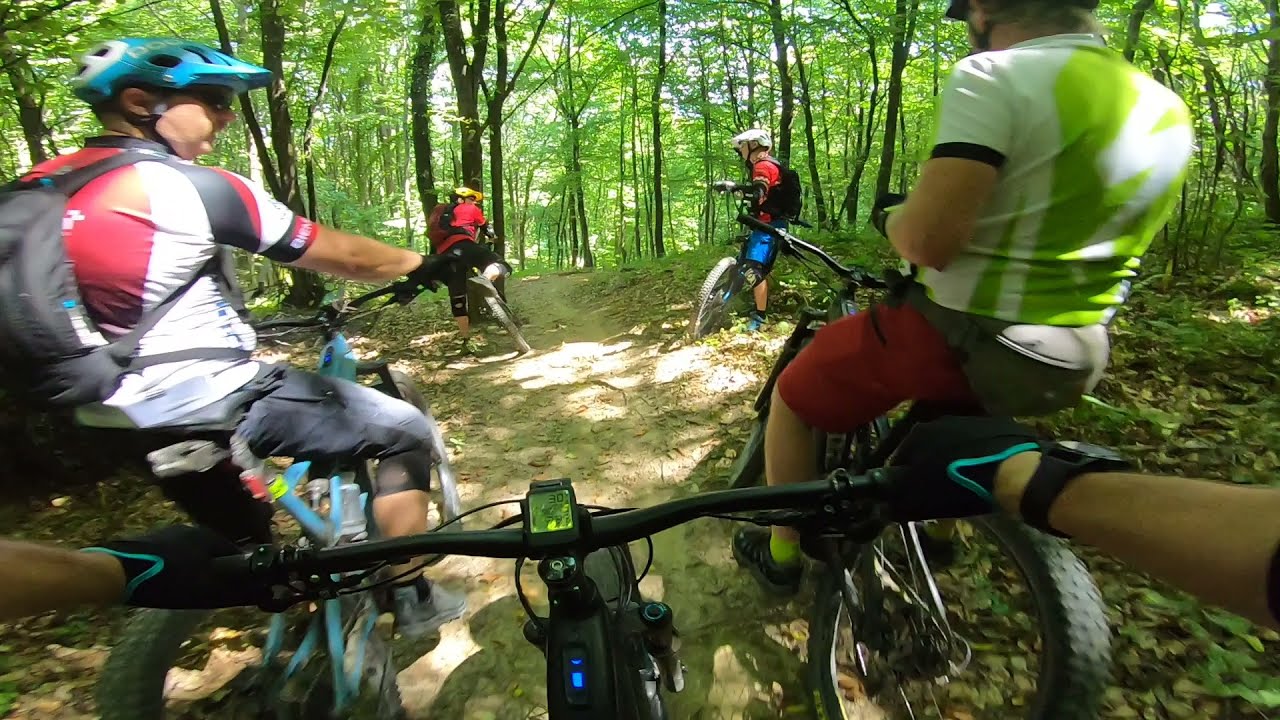Captured from the rider's perspective, likely with a helmet-mounted camera, this dynamic photo vividly portrays a group biking adventure through a lush, green forest. Dominating the foreground, the photographer's gloved hands grip the handlebars of a sleek black bicycle. Ahead, on a well-trodden dirt path encircled by towering trees, four fellow cyclists are seen resting. The trail is lined with cyclists clad in vibrant gear: the rider on the far left sports a backpack, a blue helmet, and a striking black, white, and red shirt, while adjacent to them, another wears a green and white shirt paired with red shorts. Further up the path, two more cyclists are visible, one half-seated on their bike and the other standing beside theirs, both engrossed in conversation. Each rider is well-equipped with cycling gear, including helmets and packs, set against the serene backdrop of the expansive forest.